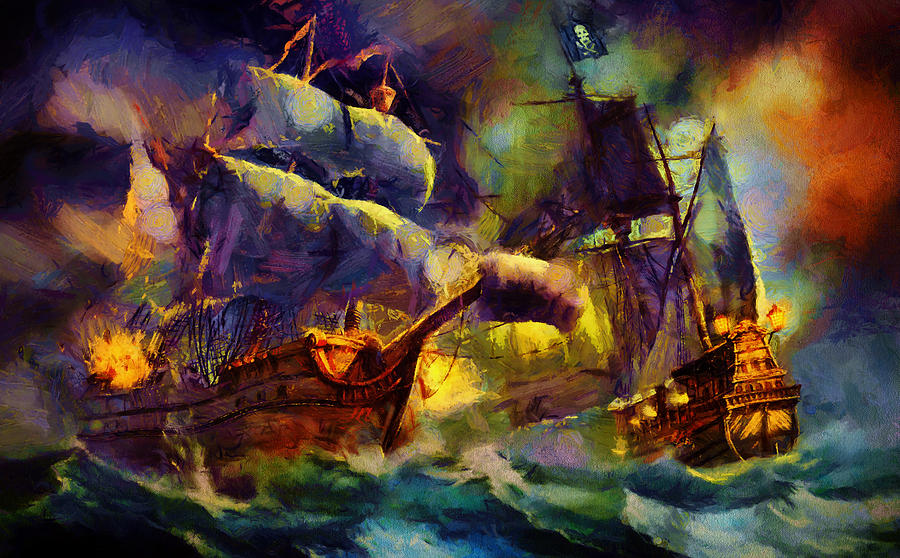This vivid painting captures a dramatic naval battle between two large, wooden ships navigating through choppy, turbulent waters. The sea churns in dark hues of blue and green, punctuated by white-capped waves, especially visible in the lower right corner. The stormy scene is set against a menacing sky, swirling with dark purples, oranges, and greens that heighten the sense of chaos and danger.

On the left, a ship with a dark orange hull and four billowing dark purple sails is engulfed in an explosion, visible as bright orange sparks—likely from cannon fire. Further enhancing the perilous atmosphere, a cannon juts out from the bow. The ship on the right, with its own dark orange body and large sails, flies a small flag adorned with a skull and crossbones at the top, indicating its pirate nature. This ship also features two lanterns on its prow and is partially obscured by the surging waves, adding to the intense action of the scene. Both vessels appear slightly tilted, as if tossed by the violent ocean, contributing to the overall impression of imminent danger and high seas adventure.